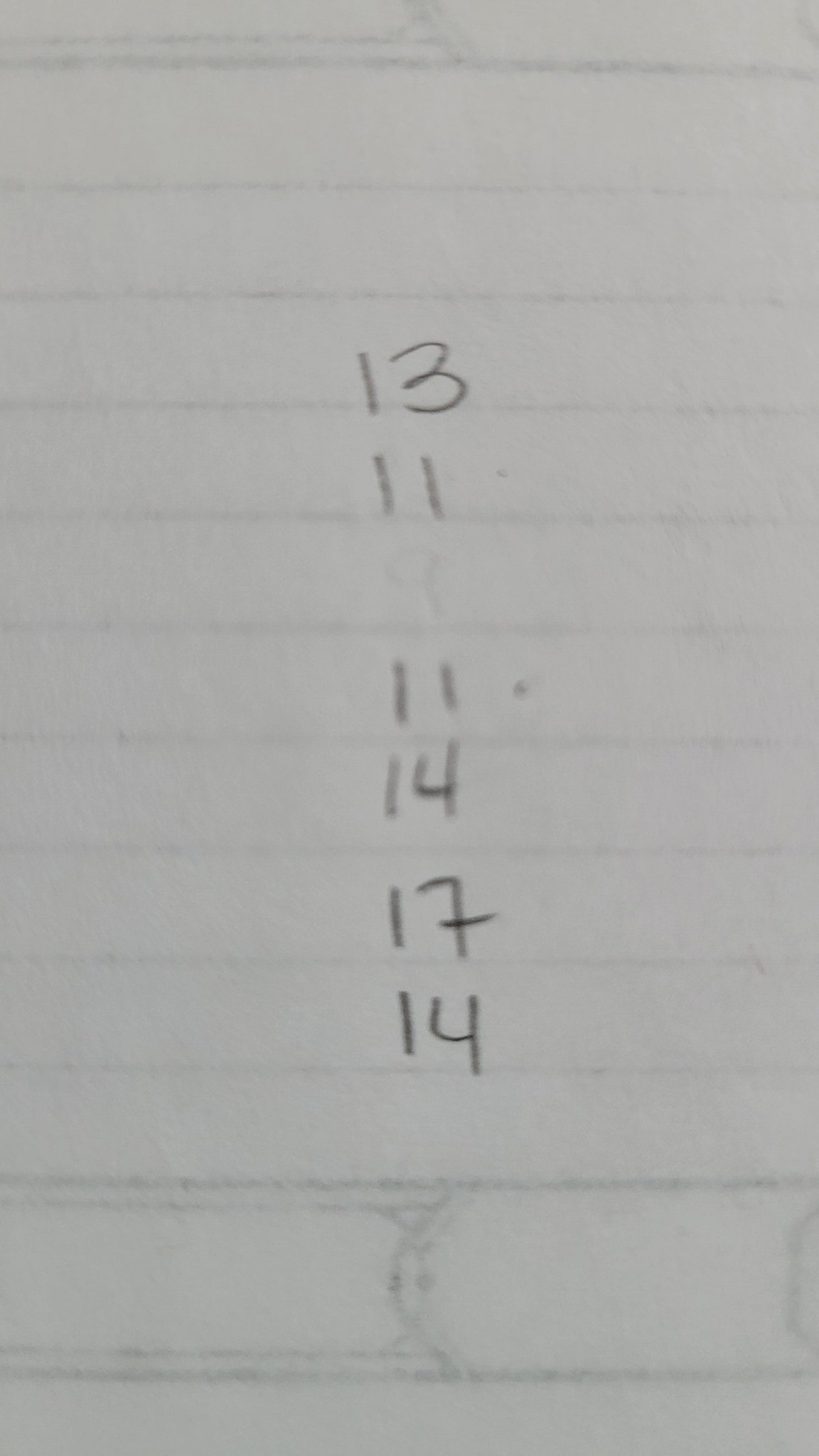The image features a sheet of faintly lined white paper, upon which are inscribed a series of numbers. At the top, the number '13' appears on the third line from the top. Below that, the number '11' is written followed by a blank space. The sequence continues with another '11', followed in succession by the numbers '14', '17', and another '14'. The remaining portion of the paper beneath these numbers is largely blank, save for a notable area where two commas are displayed, seemingly oriented in opposite directions yet almost meeting in the center of the space.